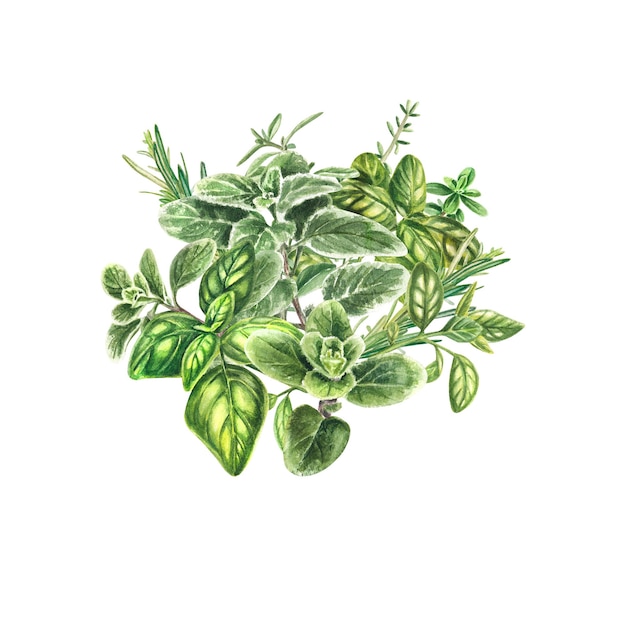This is a detailed colored pencil drawing of various green and yellow plants, drawn with a high level of realism on a white background. The composition appears to feature at least four distinct types of leaves, arranged in a visually appealing manner. The plant at the bottom has four prominent petals extending in the cardinal directions, with smaller leaves nestled at its center. To its left is a plant with bolder, slightly triangular leaves, tinged with a bright yellow-green hue and segmented by thicker white lines. At the top right, some leaves display a whitish coloration. On the far left, the leaves are similar in shape to the bottom plant but exhibit a whitish edge. Among these leaves, there are recognizable herbs such as basil, rosemary, thyme, and possibly mint, suggesting a collection of spices. The overall effect is a vibrant, professional-quality sketch that captures the intricate details of each leaf and plant.